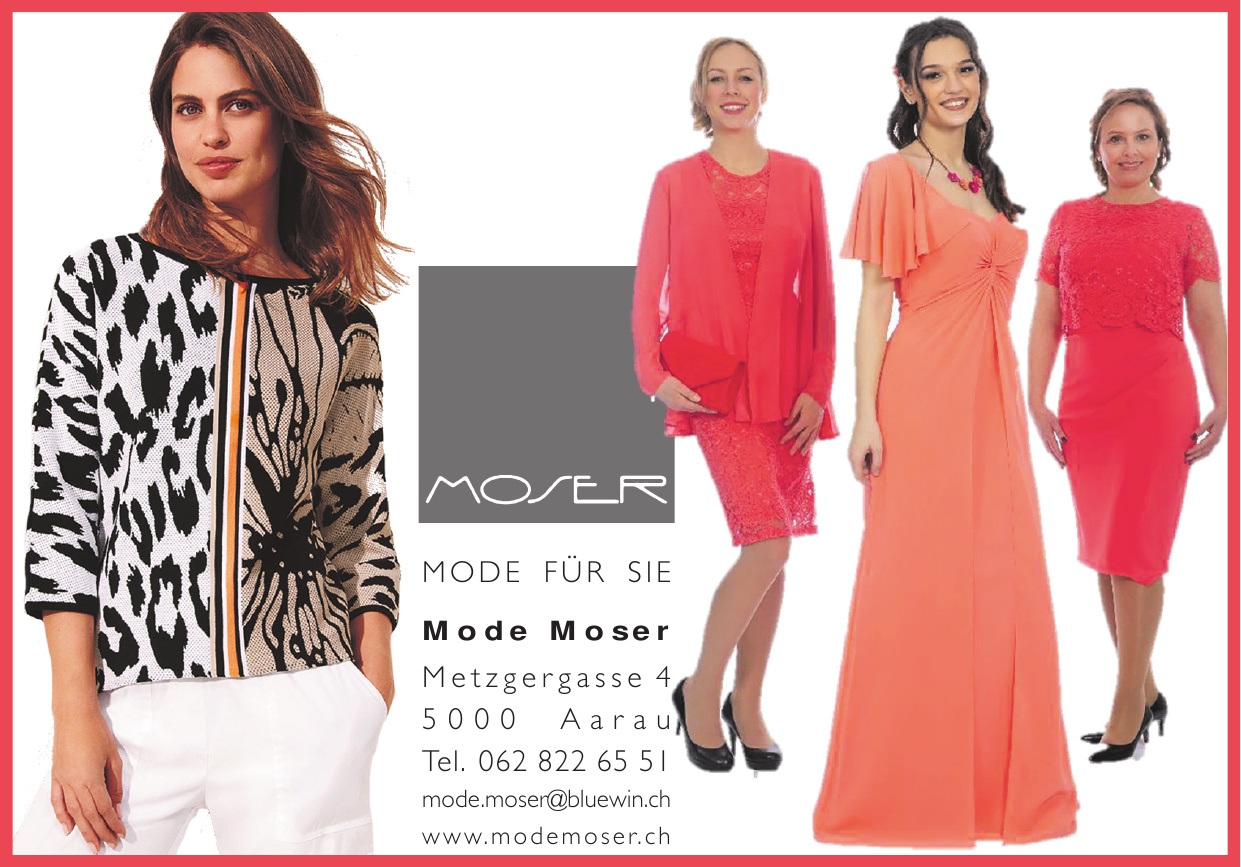This advertisement poster features a white background bordered in pink, with four women prominently displayed in photoshopped images. On the left side of the poster is a woman with long brown hair, dressed in white pants and a soft white sweater adorned with a black design resembling a flower or butterfly on the right side. To the right of her, three women are standing and posing, each wearing a dress; the dresses are colored red, orange, and red respectively. In the center-left of the image, there's a gray block containing text in white that reads "MOSER" at the top. Below that, the text says "Mode for SIE" followed by "Mode Mosser" with an address beneath, which reads "Metzgergasse 4, Aarau Tel 062 822 6551, Mod.Mosser@Bluwin.ch, www.ModMosser.ch". The colors on the poster include shades of peach, pink, white, black, orange, tan, brown, and gray, contributing to a visually appealing advertisement for the brand.